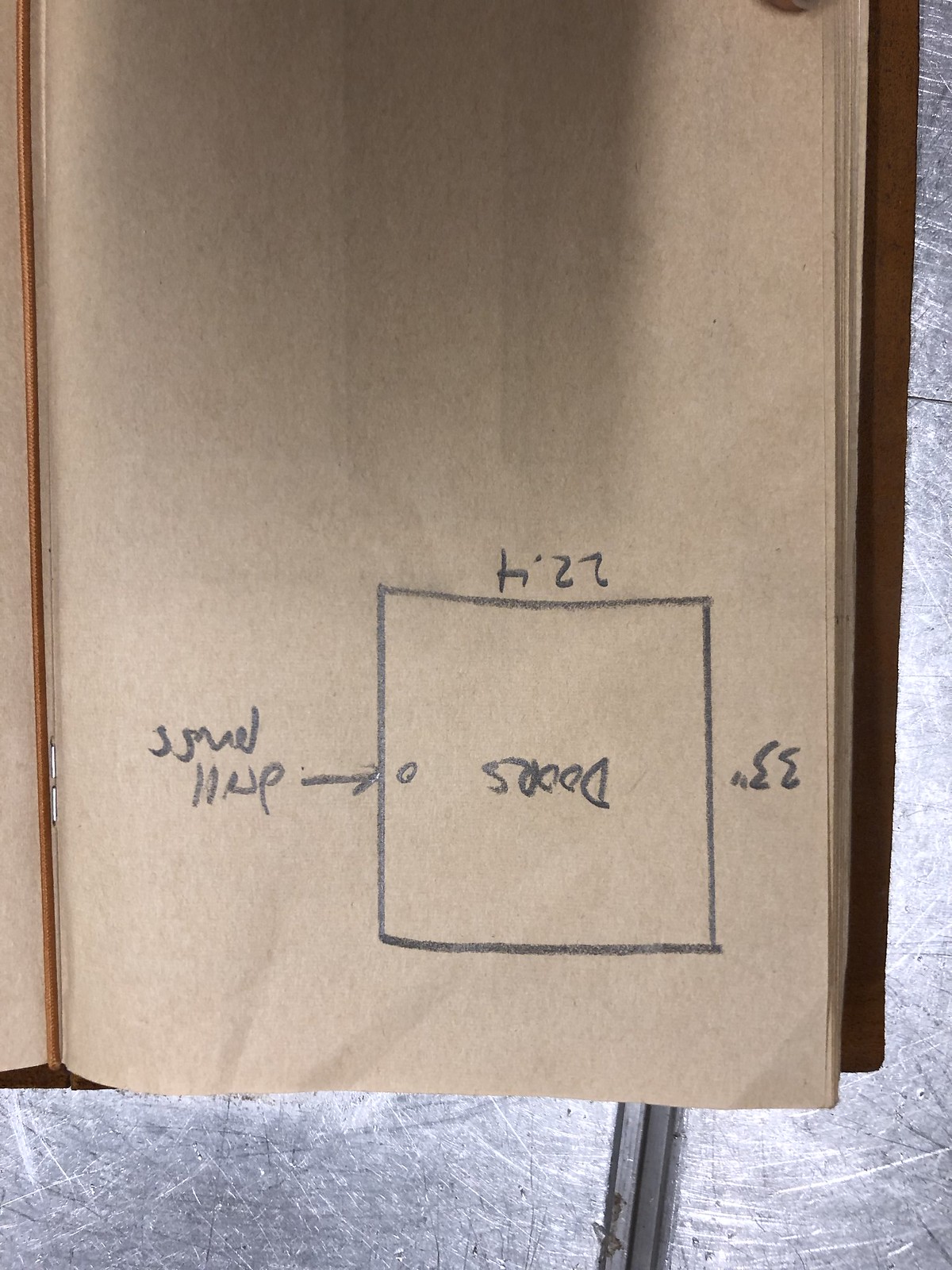This color photograph depicts an open notebook, which is flipped upside down, revealing only its right-hand page. The paper has a brown hue reminiscent of a shopping bag. The notebook lies on a reflective silver surface. Running vertically down the center of the notebook is a prominent brown line. In the top-left corner of the visible page, a neatly drawn square encloses the word "doors." Adjacent to the square, on its left side, is the notation "33 inches." On the right side of the image, the word "drill" appears, followed by another word that is indiscernible. A drawn arrow points to the right towards a small circle situated near the square’s right edge. Below the square, the figure "22.4" is written. Notably, there are no people present in the photograph, and the notebook is indeed flipped upside down.